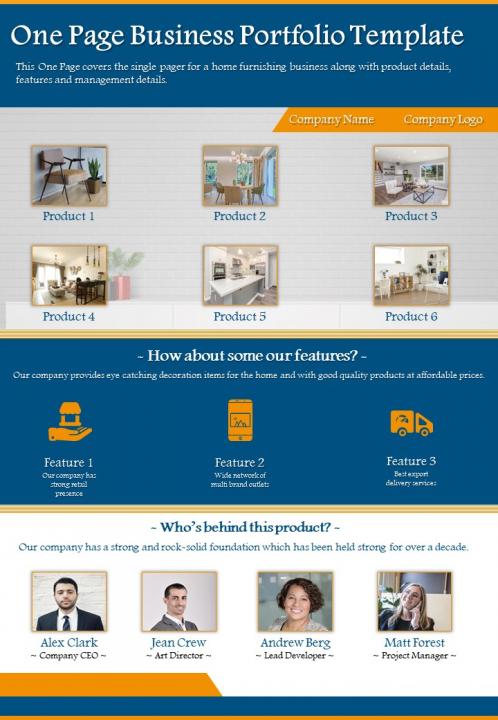Screenshot of a One-Page Business Portfolio Template for a Home Furnishing Business

The screenshot features a website design template labeled "One-Page Business Portfolio Template" at the top. The header is a blue bar with white text, highlighting the simplicity and elegance intended for a home furnishing business. The section below the header includes essential product and management details.

On the top right, there's an orange bar displaying the company name and logo against a grey background. This section includes placeholders for six product images labeled "Product 1" through "Product 6," reflecting the potential visual representation of the company's offerings.

Further down is a blue section outlined in yellow, prompting visitors with the text "How about some of our features." This section highlights three key features of the business, each represented by an orange icon in the center, making it visually appealing and easy to understand.